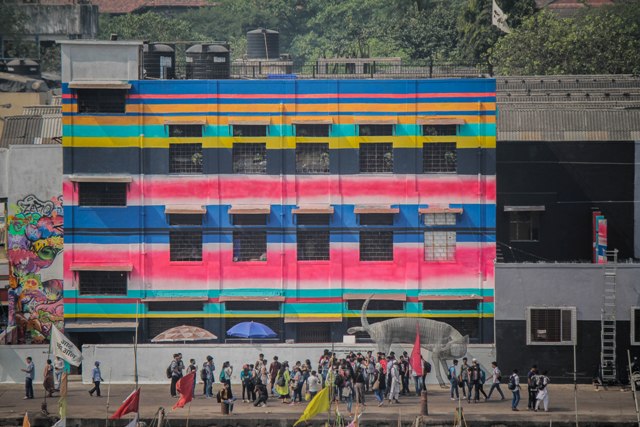This is an image of a vibrant, three-story building, possibly a school, with a striking and colorful mural adorning its side. The mural comprises horizontal stripes in an array of vivid colors, including blue, pink, orange, light blue, yellow, black, white, and green. These stripes vary in thickness, creating a mesmerizing pattern across the entire facade. On the far right side of the building, the colors shift primarily to black and gray tones.

At the top of the building, there is a flag, and the structure features a balcony. Behind the building, trees can be seen, adding a touch of nature to the urban scene. 

The mural also contains intricate details, such as people walking—some holding flags, one pink and one white—and people with umbrellas. Among the vibrant colors at the bottom of the mural, there's a depiction of a cat bending and looking back at the crowd, adding a whimsical touch to the scene. The left-hand side of the mural features a plethora of colorful doodles and drawings.

In front of the building is a crowd, which appears to be children with backpacks, possibly indicative of a school environment. The scene gives an impression of a lively protest or assembly, adding a dynamic human element to the colorful backdrop of the mural.